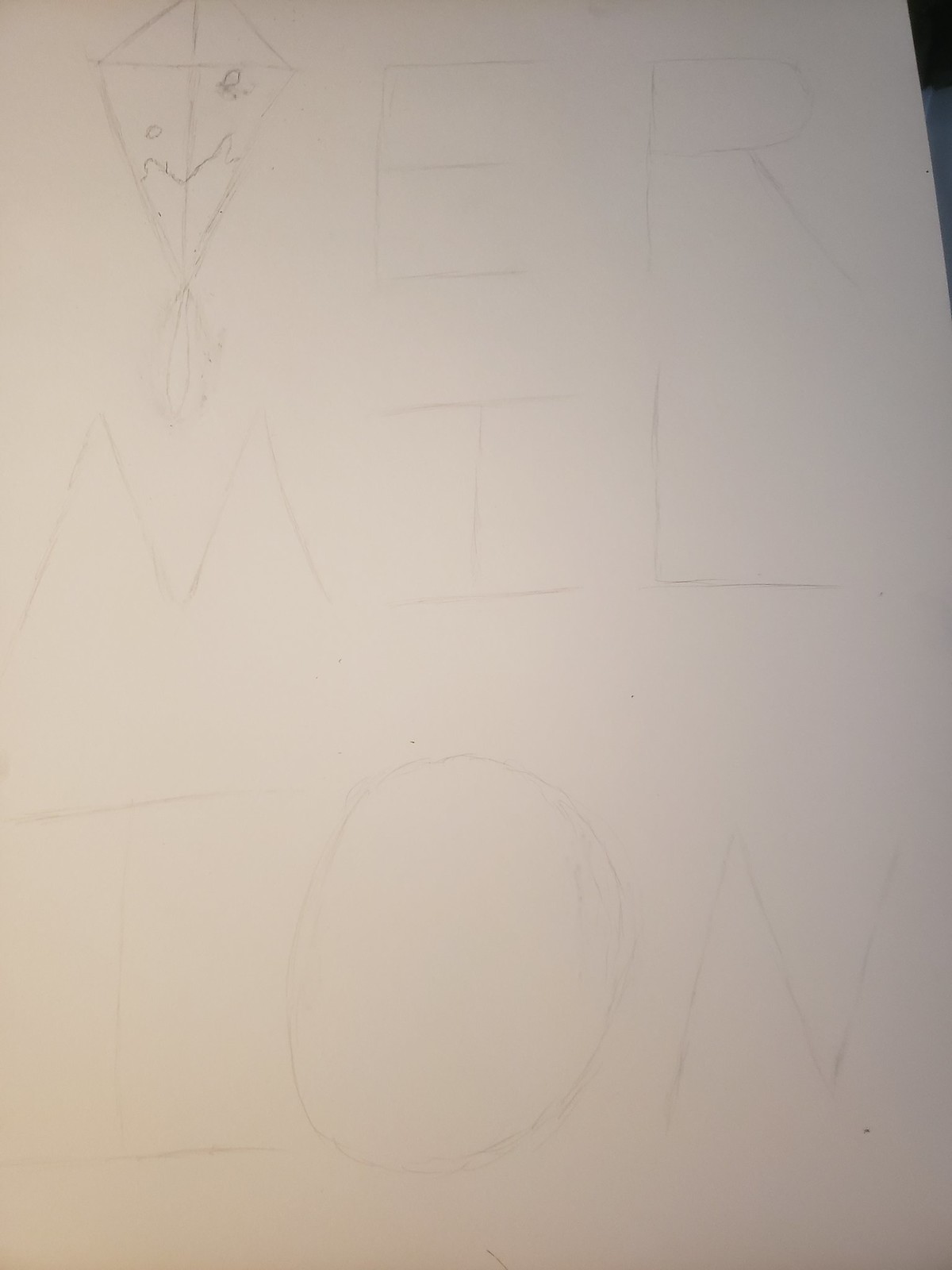This is a color photograph of a very large white sheet of paper that takes up most of the image. The faint sketches and outlines suggest the paper extends beyond the visible frame. The lighting is uneven; it is better towards the left middle and darker in the upper right corner, where a small sliver of black and gray edges past the paper. In the top left corner, there is a simple pencil drawing of a kite—outlined in a diamond shape with a small tail. To the right of the kite, there are capital letters “E” and “R.” Below these, in similarly faint writing, are the letters “M,” “I,” and “L.” At the bottom, the larger but equally light letters "I," "O," and "N" can be seen. Despite the image being black and white, one caption suggests the possibility of the letters forming the word "Vermillion." The overall impression is that it might have been drawn by a child, given the simplicity and light touch of the sketches and letters.